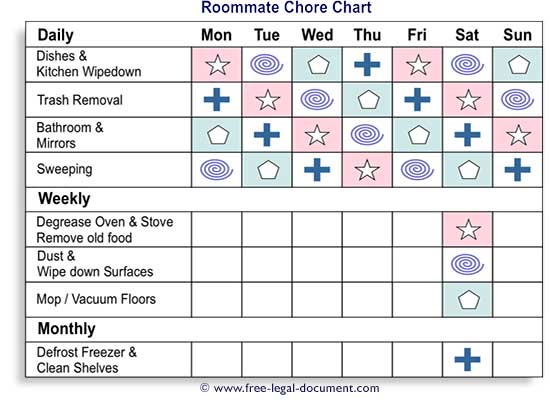The image depicts a structured Roommate Chore Chart with a white background, divided by black lines into several categories and areas for daily, weekly, and monthly tasks. The title "Roommate Chore Chart" is prominently displayed in dark blue and centered at the top. 

On the left-hand side of the chart, there are three main subheadings: "Daily," "Weekly," and "Monthly," each printed above corresponding rows of chores. The "Daily" section includes tasks such as dishes and kitchen wipe down, trash removal, bathroom and mirrors, and sweeping. The "Weekly" section lists chores like degreasing the oven and stove, removing old food, dusting and wiping down surfaces, and mopping/vacuuming floors. The "Monthly" section has a single item: defrosting the freezer and cleaning shelves.

Across the top of the chart are the days of the week, from Monday to Sunday, abbreviated as MON, TU, WED, THU, FRI, SAT, and SUN. Each day has a box that includes one of several symbols, such as a white star on a pink background, a blue swirl on a white background, a white pentagon on a teal background, or a blue cross on a white background. These symbols are used to allocate chores to different roommates, indicating who is responsible for each task on a given day.

The chart is meticulously organized to ensure chores are evenly distributed among roommates, visually guiding each person to complete their assigned responsibilities efficiently.